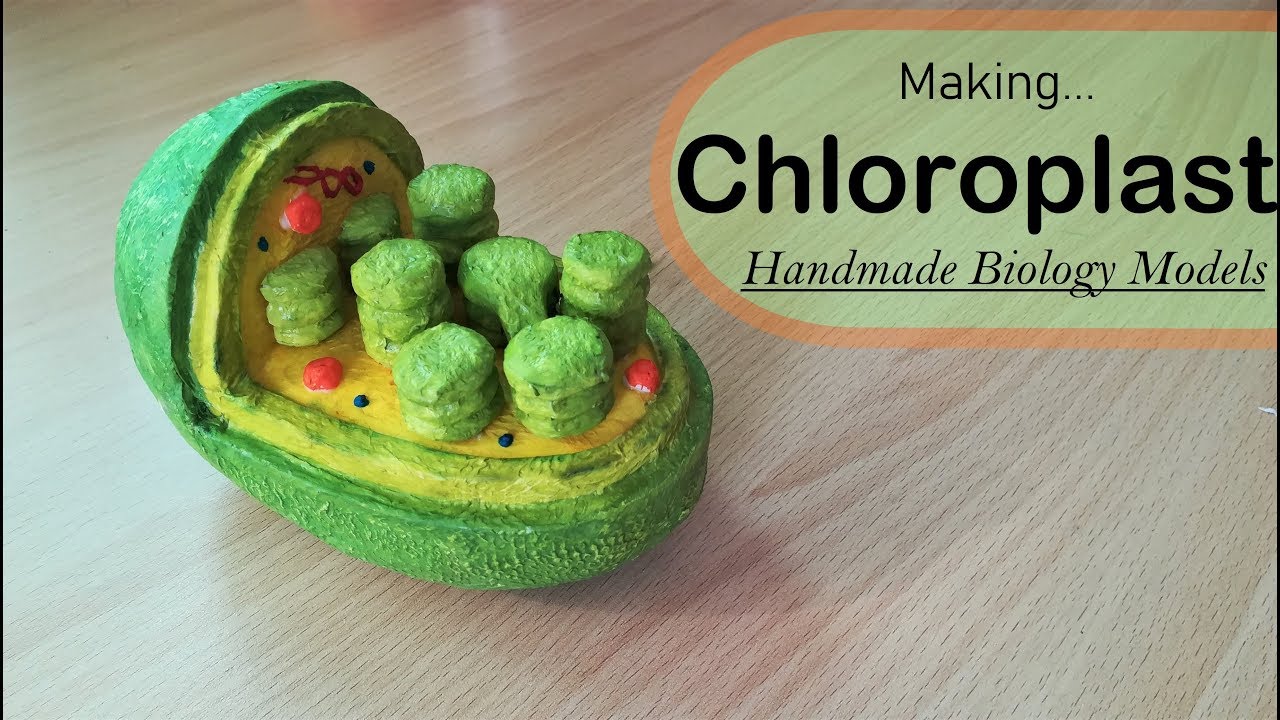The landscape-oriented photograph showcases a handmade biology model of a chloroplast placed on a light faux-wood surface with medium brown diagonal wood grains. The focal point of the image is an intricately crafted, ceramic representation of a chloroplast that resembles a partially cut avocado or lime. The model features an outer green layer with a quarter section removed to reveal the lime-green and yellow interior. Inside the yellow core, there are multiple green cylindrical structures stacked on top of each other, interspersed with small red and black dots. In the upper right corner of the image, a label on a pinkish-orange background with black bold text reads, "Making... Chloroplast... Handmade Biology Models." The entire arrangement allows viewers to visually explore the detailed inner layers and components of the chloroplast model.